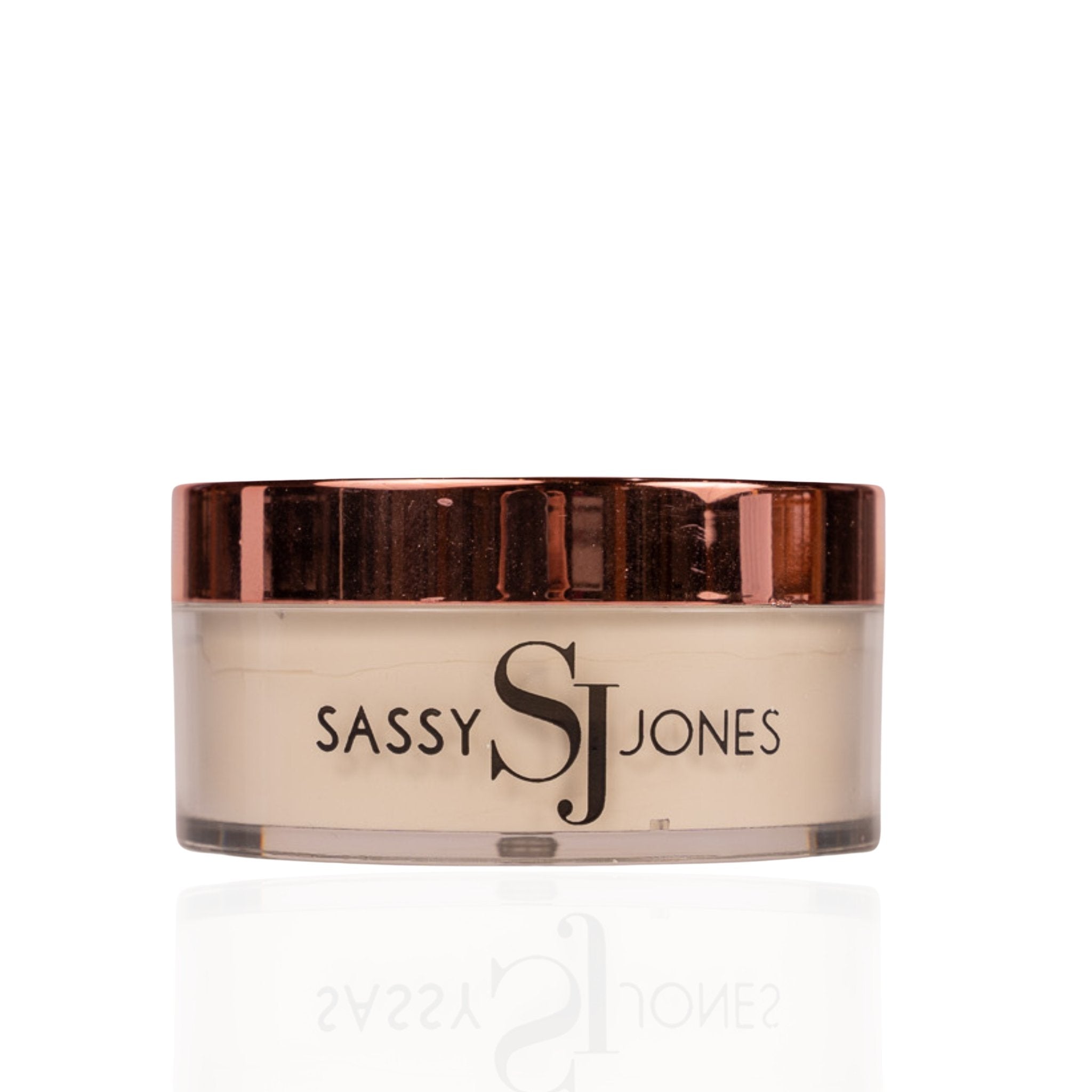The photograph features a small, cylindrical jar, measuring roughly 2 to 3 inches in height, prominently displayed against a white background. The jar, likely containing translucent powder or moisturizer, has a clear glass body that reveals a white substance inside. Its design includes a distinctive copper or gold metallic lid that is highly reflective, capturing reflections of windows, doors, and shadows. The branding on the jar reads "SASSY S.J. JONES," with "SASSY" and "JONES" in dark, all-capital letters, and "S.J." presented in a larger, ornate font, positioned slightly lower than the preceding text. This reflective base allows the label to be seen in reverse, underscoring the jar's polished and new appearance.